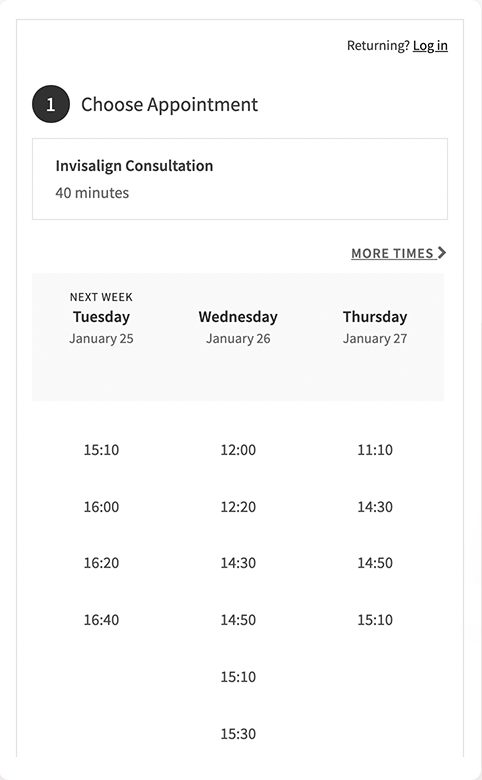This image is a screenshot from a phone displaying an appointment scheduling page. The screenshot lacks a defined outer border but features a thin grey frame, enclosed within a thinner, rectangular portrait border on a white background. At the top left corner, the text "Returning" appears next to an underlined "Login," both in black. Below, a black circle with a white number "1" indicates the first step: "Choose Appointment," also in black text.

Beneath this, a thin grey rectangle in landscape orientation reads "Invisalign Consultation - 40 minutes." Directly below, there's an option to "Select More Times" marked with a right caret.

The next section presents appointment dates and times. For the following week, the available dates are Tuesday, January 25th, Wednesday, January 26th, and Thursday, January 27th. Each date lists specific time slots: 

- Tuesday offers appointments from 10:15 AM to 6:40 PM.
- Wednesday's slots range from 10:00 AM to 3:30 PM.
- Thursday has appointments available from 11:10 AM to 3:10 PM.

Users can select an available time slot to proceed to the next step in booking their appointment.